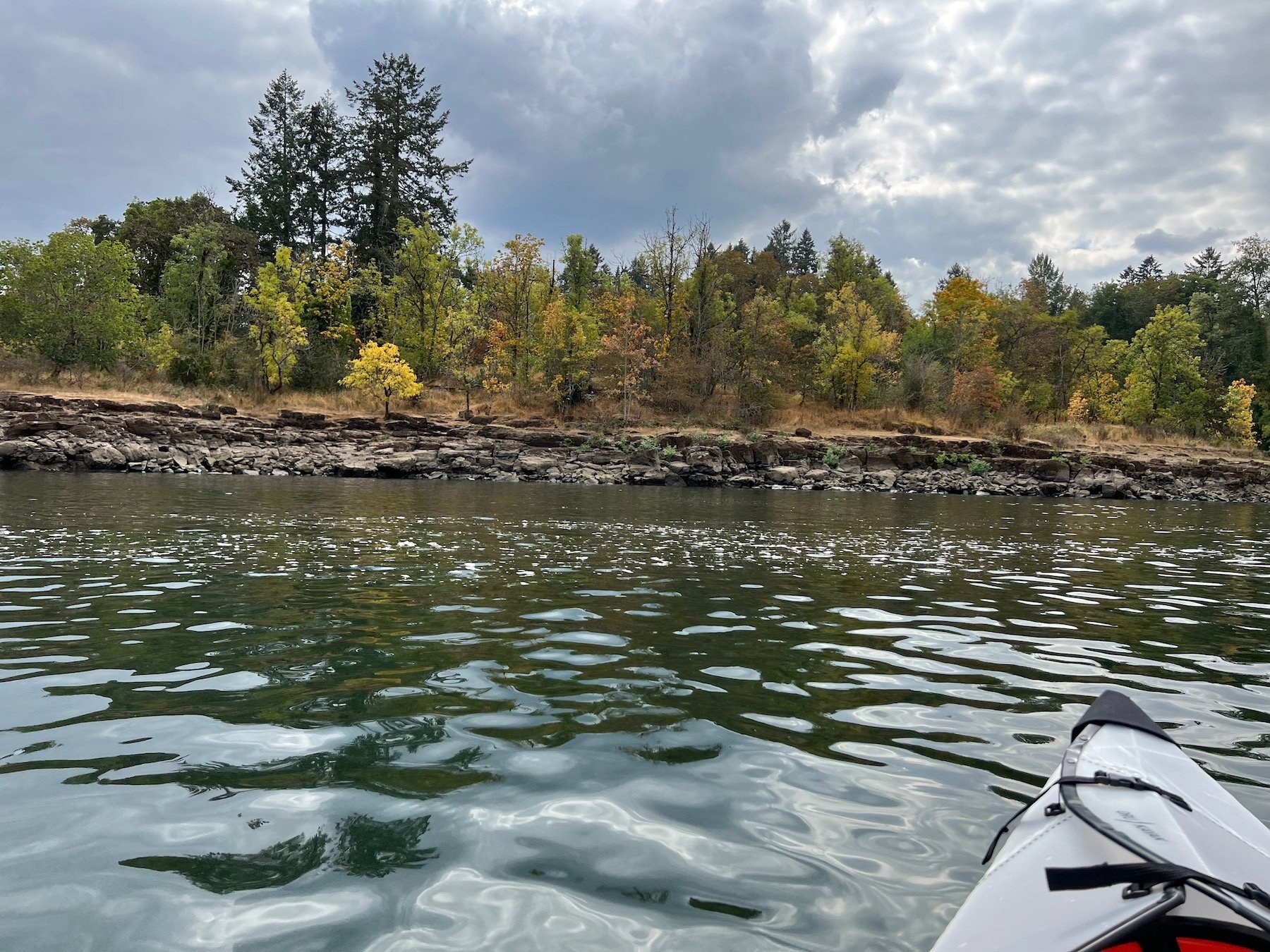The image is a photograph captured from the perspective of a person kayaking on a calm river or lake. In the bottom right corner, the tip of the white kayak, which tapers to a point and slightly curves upward, is visible. The water, placid and greenish, reflects the surrounding vegetation. Directly in front of the camera lies a shoreline featuring a partially crumbling rocky cliff, only a few feet high, topped with an embankment densely covered in trees. The foliage is in various stages of autumn, with leaves turning yellow and orange. The sky overhead is heavily overcast with gray clouds, contributing to the cool and peaceful ambiance. The natural landscape is serene, with no other people or animals in sight, emphasizing the solitude of the kayaker.